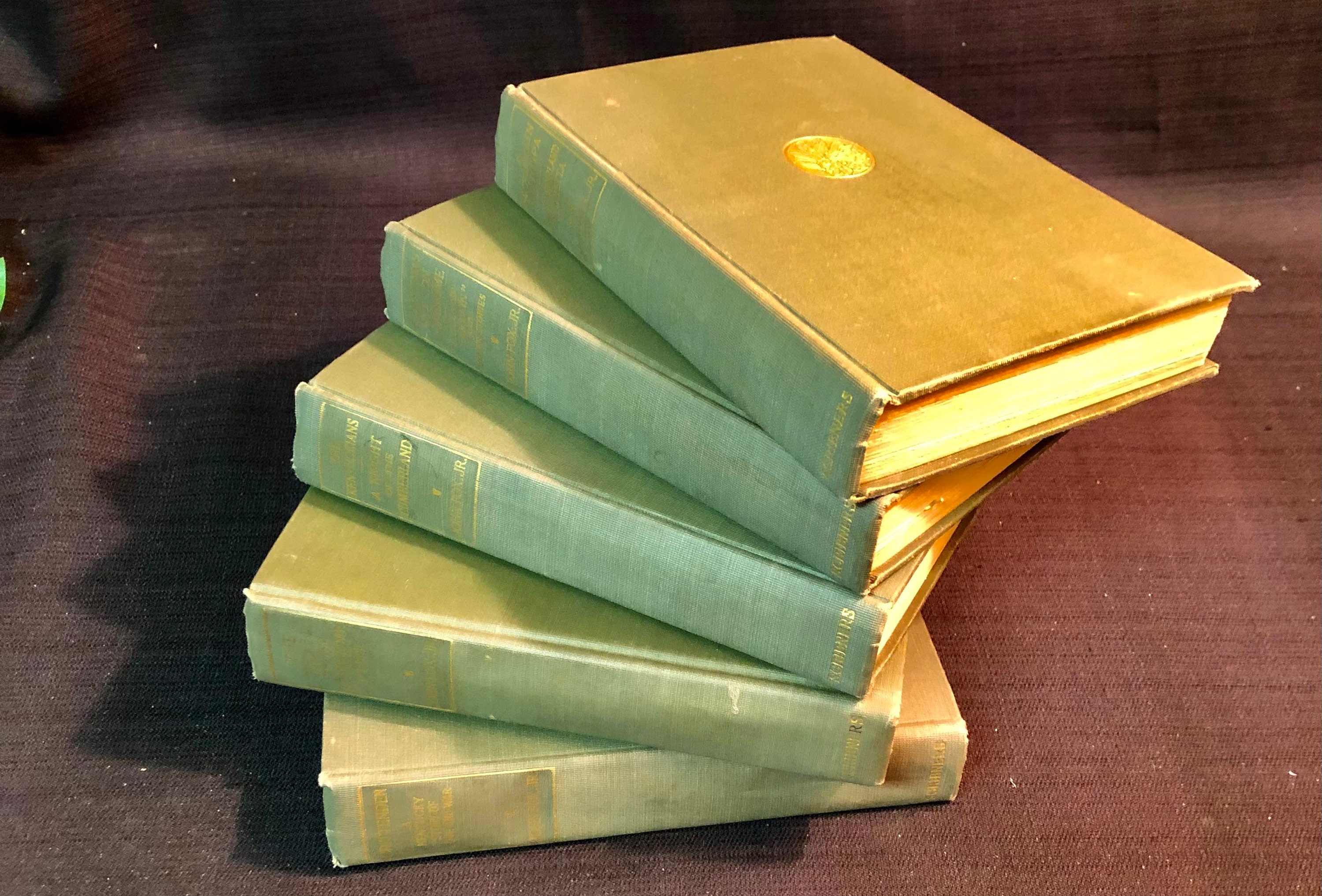The photograph features a neatly arranged stack of five books, artfully positioned in a stair-like or swivel staircase fashion, creating an intriguing visual effect. The books, primarily light green, likely appear so due to the right-side light source casting a warm, yellowish glow. Each book is approximately one and a half inches thick and bound in hardcover. The book at the top prominently displays its front cover, which features a striking golden circular disk in the center. This stack sits atop a dark, richly textured fabric, which could be a tablecloth or carpet, boasting a deep hue of dark purple or wine red. Shadows cast to the left emphasize the directional lighting and add depth to the scene, enhancing the educational and reading ambiance.